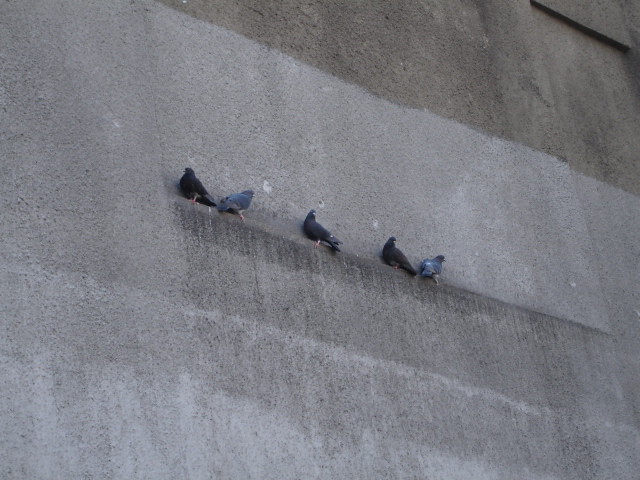This photorealistic image depicts a concrete wall with a narrow, uneven ledge that appears almost imperceptible from the viewer's perspective. The ledge is part of a cement wall, likely unintended and possibly the result of imperfections or patchwork, as indicated by the varying shades of gray in the wall. There are five pigeons sitting on this ledge. The first pigeon, a black one, is positioned towards the left center and faces left. Next to it is a gray pigeon facing right. A darker gray pigeon occupies the center, with its body oriented left and head turned to the right. To the right of this central pigeon, another darker gray pigeon mirrors the previous pigeon’s pose. Lastly, a light gray pigeon on the far right faces right. The concrete wall displays a noticeable color difference, with lighter gray cement on the lower portion and darker cement in the top right corner, suggesting either replacement or inconsistencies in the wall’s construction.